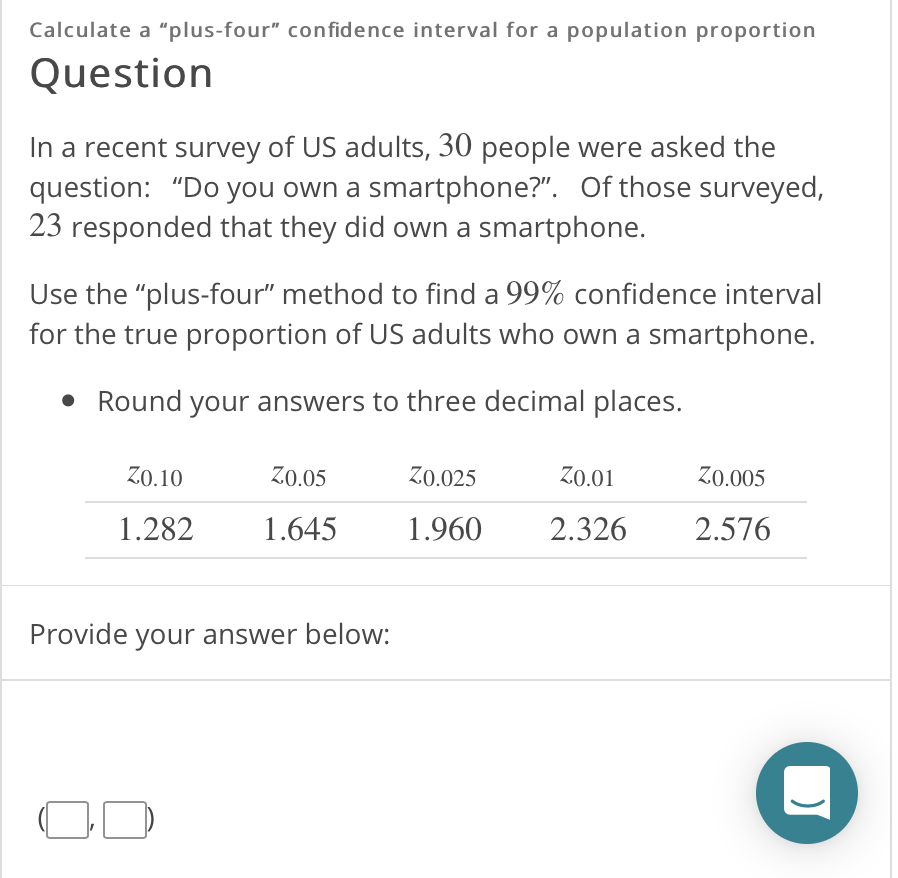**Caption:**

The image illustrates a test question about calculating a "plus-4" confidence interval for a population proportion. The question is prominently displayed in bold black letters and states: "In a recent survey of US adults, 30 people were asked if they own a smartphone, with 23 responding affirmatively. Use the plus-4 method to find a 99% confidence interval for the true proportion of US adults who own a smartphone. Round your answers to three decimal places."

Below the question, a table lists z-values corresponding to various significance levels:

- z(0.10): 1.282
- z(0.05): 1.645
- z(0.025): 1.960
- z(0.01): 2.326
- z(0.005): 2.576

A light gray line separates the z-values from additional numerical data, although the exact numbers and their purpose are not specified in the description.

Further down, another light gray line precedes an input box prompting for the answer: "Please provide your answer below." This section features a bracket followed by two plain boxes separated by a comma, indicating where the interval limits should be entered.

To the far right of the image, a white speech bubble with a bluish-green smile and surrounded by a matching bluish-green circle provides a friendly, encouraging touch to the question setup.